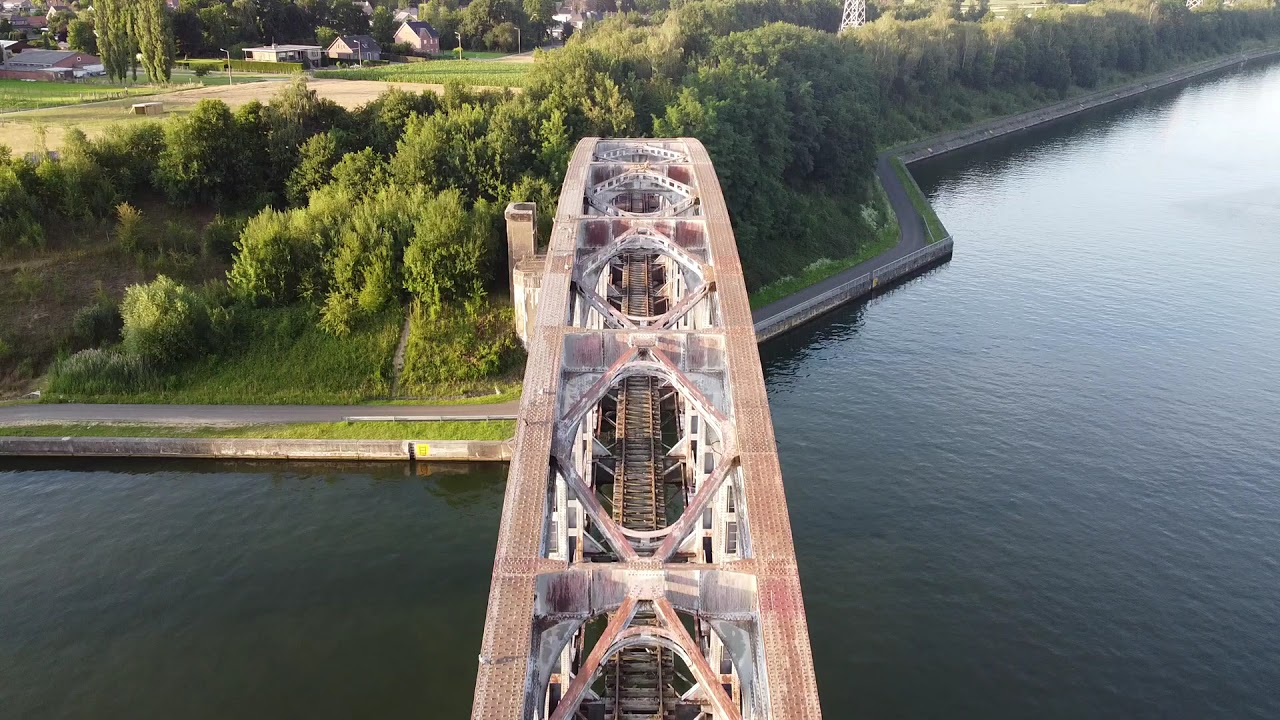This aerial photograph captures a striking trestle bridge spanning a body of water, possibly a lake. The bridge structure features a mix of reddish-bronze, white, and light gray crisscross braces, with a set of grayish-red train tracks extending down its center. The water underneath shimmers in shades of dark greenish-blue. Flanking the bridge are well-maintained concrete sidewalks and light posts. Beyond the bridge, lush green scenery unfolds with thick woodlands of dark green trees, manicured grass fields, and a residential neighborhood featuring various one-story and two-story homes with dark roofs. The image encapsulates the harmonious blend of natural beauty and architectural design.